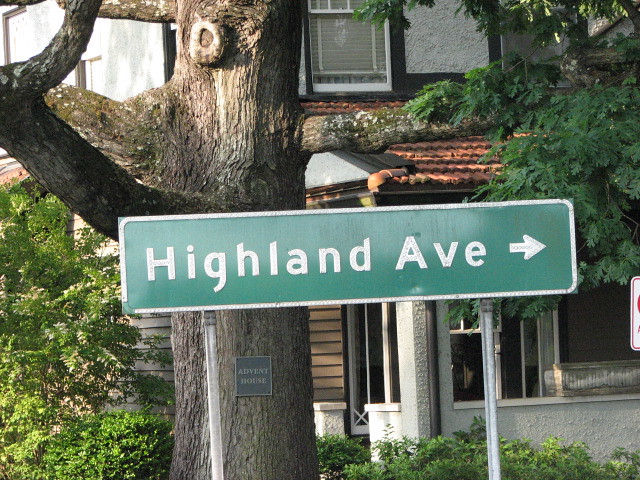This outdoor daytime photo captures a detailed scene centered around a green, rectangular street sign mounted on two metal poles. The sign prominently displays "Highland Ave" in white lettering with an arrow pointing to the right. In the foreground, a large, ancient tree with ashy bark and moss hosts a small black plaque with bronze colored letters that read "Advent House." Behind the tree, a two-story house is partially visible. The house features a red terra cotta roof over the porch and a mix of brown clapboard siding on the lower floor and off-white stucco on the upper floors. One of the windows, framed with dark brown casing, can be seen alongside some surrounding trees and greenery.